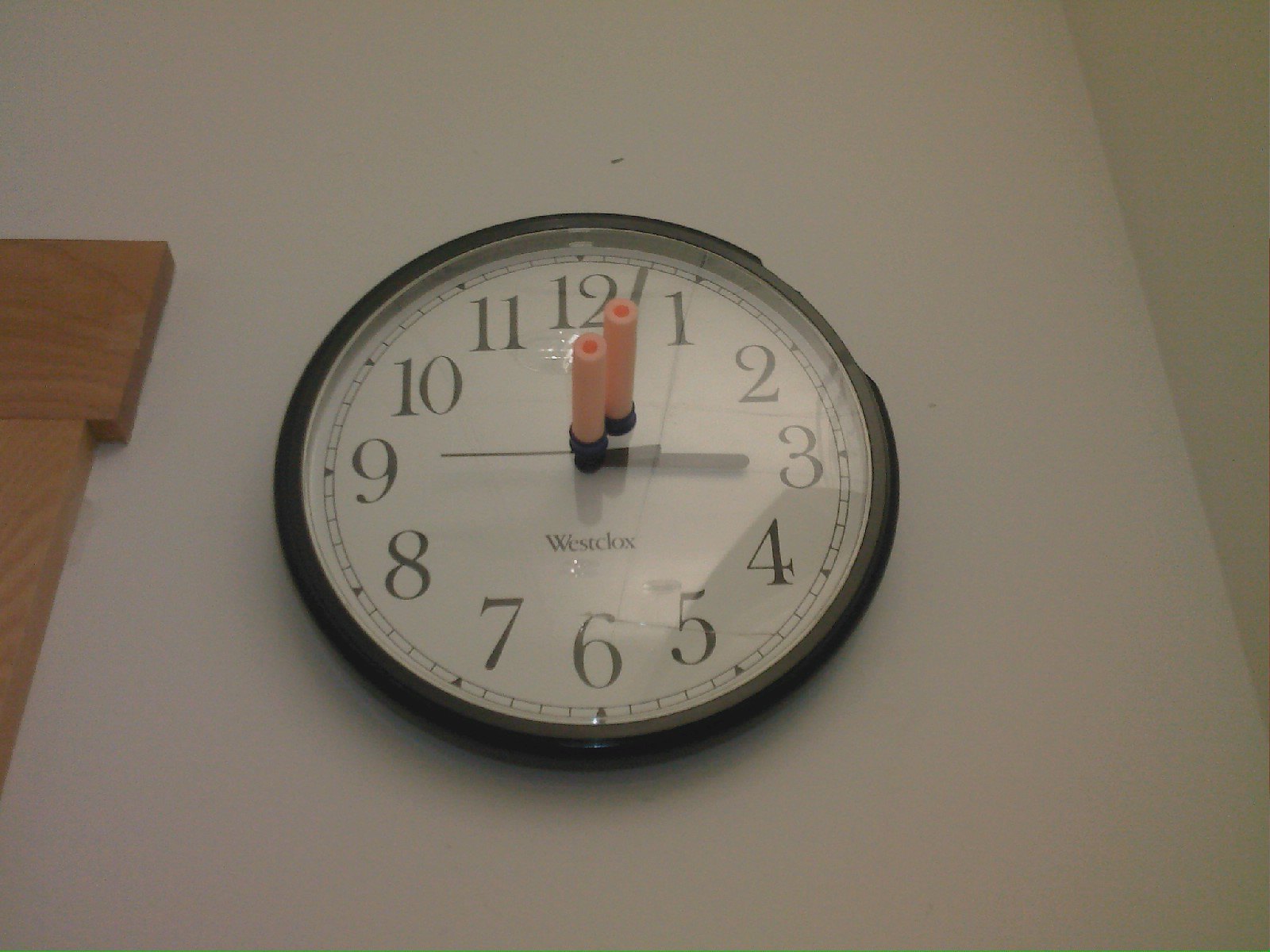In this image, we see a clock mounted on an off-white wall, with visible wood trim off to the left. The clock has a white face adorned with black numbers indicating the hours from 1 to 12, and the words "Westclox" are printed just above the 6. The hands of the clock are positioned to show the time as three minutes past three, with the larger minute hand on the 3-minute mark, the shorter hour hand on the 3, and the slim second hand pointing at the 9. The face of the clock is protected by a glass cover, and two black suction cup darts with purple tubing are stuck to the middle of the glass. The black plastic rim around the clock's face is chipped on the top right, indicating previous damage. The wall behind the clock is not completely visible, but its off-white hue contrasts with a wooden board that extends partway across the wall to the left, possibly hinting at the presence of a doorway.